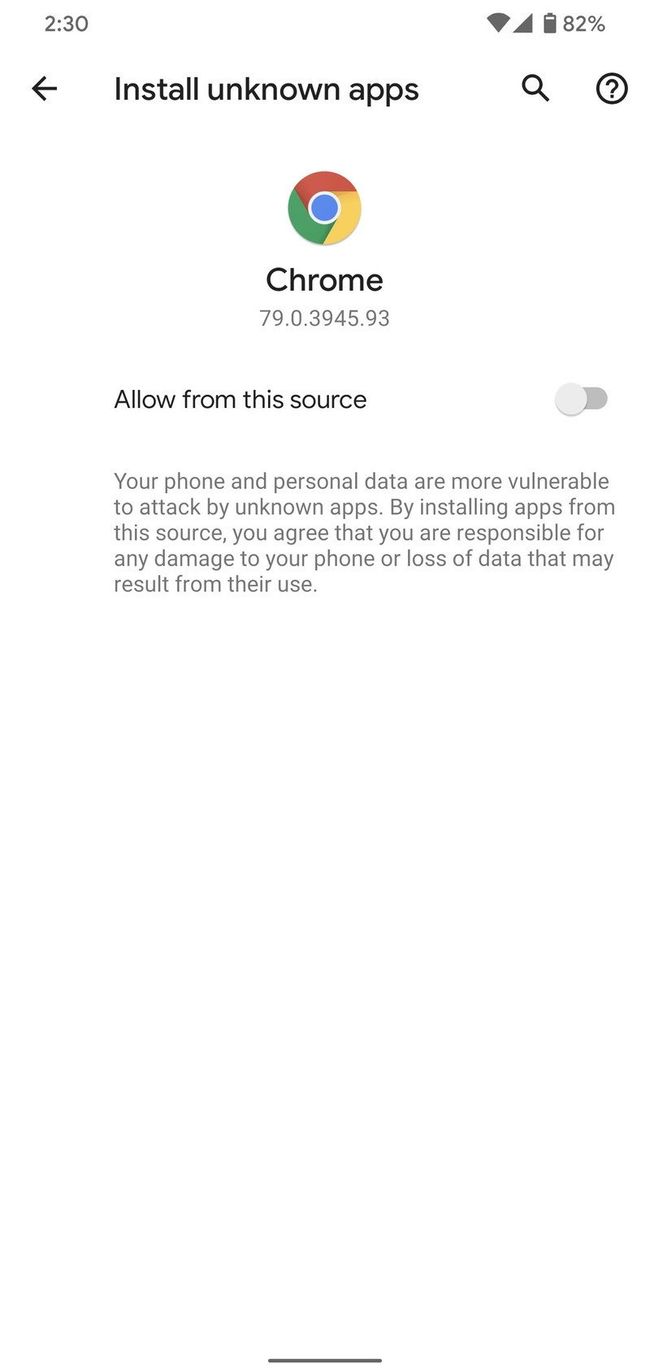The image depicts a screenshot of a smartphone's settings page for the Chrome browser. At the top, the Chrome icon is prominently displayed, consisting of a blue circle surrounded by white, with outer segments in red, green, and yellow. The title "Chrome" is written in black text beside the icon, followed by the version number "79.0.3945.93."

Below the title, there is a line of black text stating, "Allow from this source." To the right of this text, a slider switch is shown; it is currently in the "off" position, indicated by a gray circle and a gray line. The circle is positioned to the left side, signifying that the slider is inactive.

Further down, a warning message in gray text reads, "Your phone and personal data are more vulnerable to attack by unknown apps. By installing apps from this source, you agree that you are responsible for any damage to your phone or loss of data that may result from their use." The bottom of the image features a white background with a short gray line at the very bottom edge, hinting at the interface design.